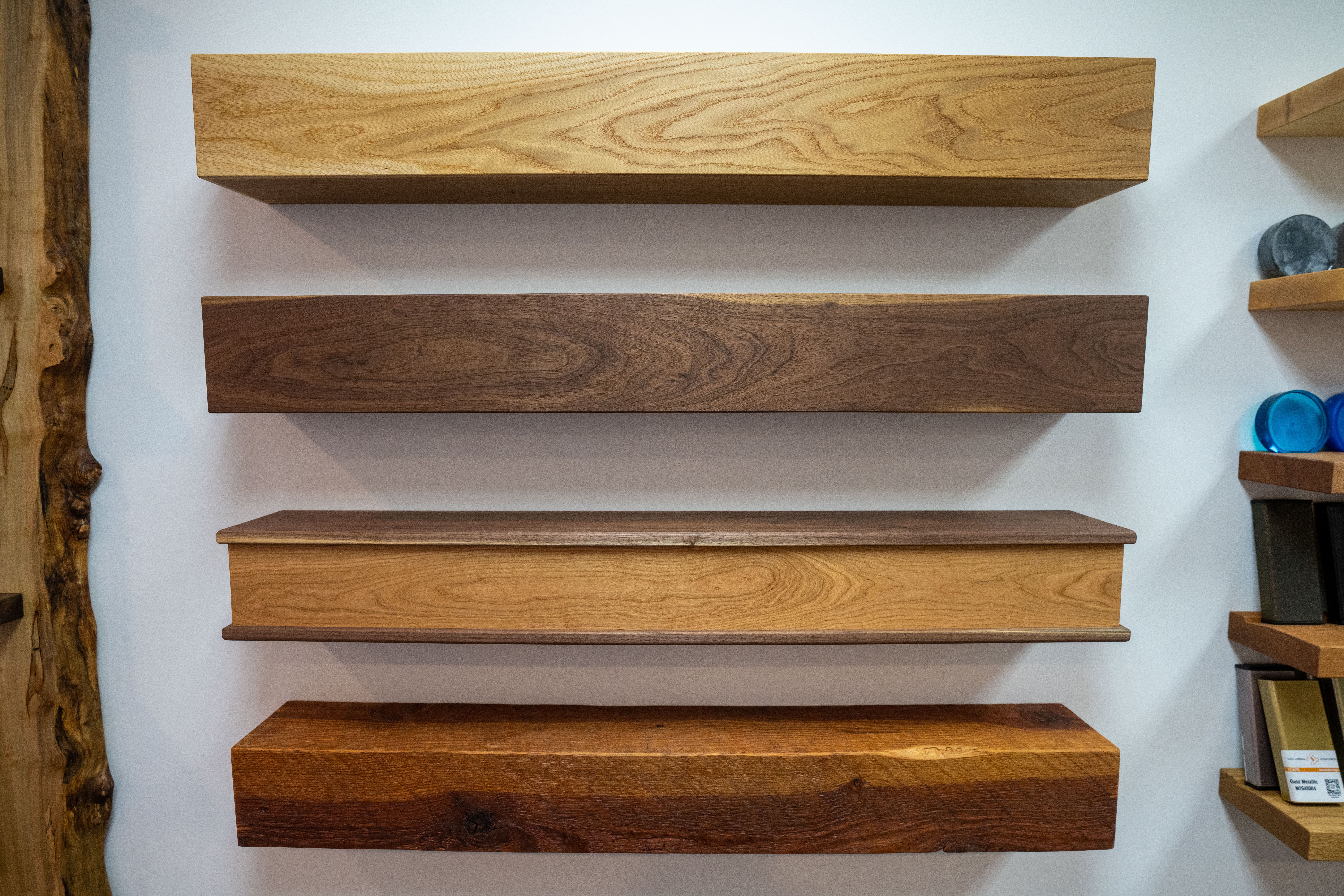The image is a color photograph in landscape orientation, showcasing a display of four wooden shelves on a white wall. Each shelf, which might also be described as mantles, exhibits a unique wood grain and staining, varying from light honey to dark browns. The shelves are aligned horizontally, one above the other, and occupy most of the image's width, with uniform spaces between them. 

From top to bottom:
1. The top shelf features a light honey-colored wood grain.
2. The second shelf exhibits a darker brown stain with visible wood grain.
3. The third shelf has a dark brown top and bottom with a light honey side panel facing outward.
4. The bottom shelf displays a two-tone design, light on the top and dark on the bottom.

On the left side of the image, there's a vertical segment of wood with a natural live edge. On the right, partially visible, are several narrower shelves, some of which have objects stacked on them, including a blue object on the second shelf from the top. The style of the photograph is representational realism, capturing the textural details and varying hues of the wooden elements.